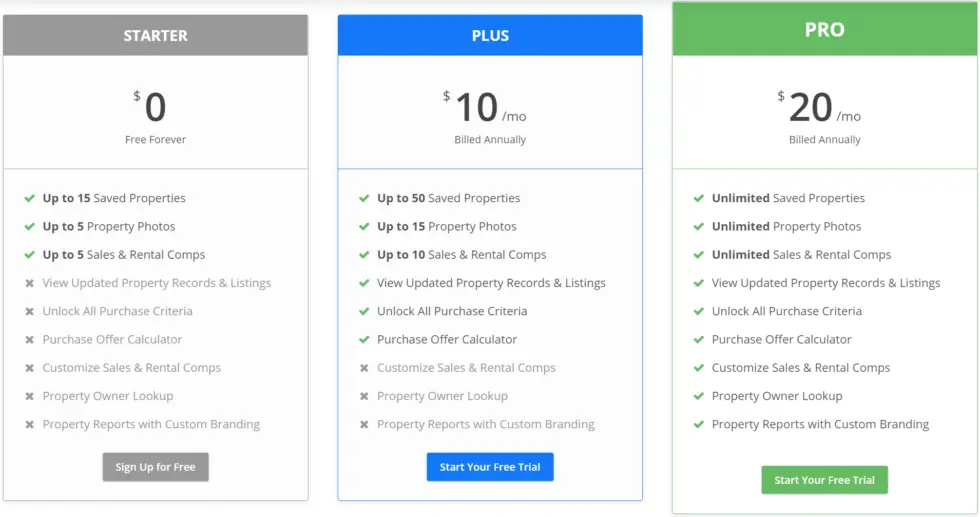This image depicts a webpage offering three subscription plans for a property management service. Each plan is outlined with its features and pricing options.

1. **Starter Plan**: 
   - **Cost**: Free
   - **Features**: Includes up to 15 saved properties, up to 5 property photos, and up to 5 sales and rental comparisons.
   - **Sign-Up**: A "Sign Up for Free" button is available at the bottom of this plan.

2. **Plus Plan**: 
   - **Cost**: $10 per month, billed annually
   - **Features**: Offers up to 50 saved properties, up to 15 property photos, up to 10 sales and rental comparisons, updated property records and listings, access to all purchase criteria, and a purchase offer calculator.
   - **Sign-Up**: A "Start Your Free Trial" button is provided at the bottom.

3. **Pro Plan**: 
   - **Cost**: $20 per month, billed annually
   - **Features**: Provides unlimited saved properties, unlimited property photos, unlimited sales and rental comparisons, updated property records and listings, access to all purchase criteria, a purchase offer calculator, customized sales and rental comparisons, a property owner lookup, and property reports with custom branding.
   - **Sign-Up**: A "Start Your Free Trial" button is available at the bottom.

The Starter Plan includes a "Sign Up for Free" button, while both the Plus and Pro Plans feature a "Start Your Free Trial" button, encouraging users to test the service before committing to a paid subscription.